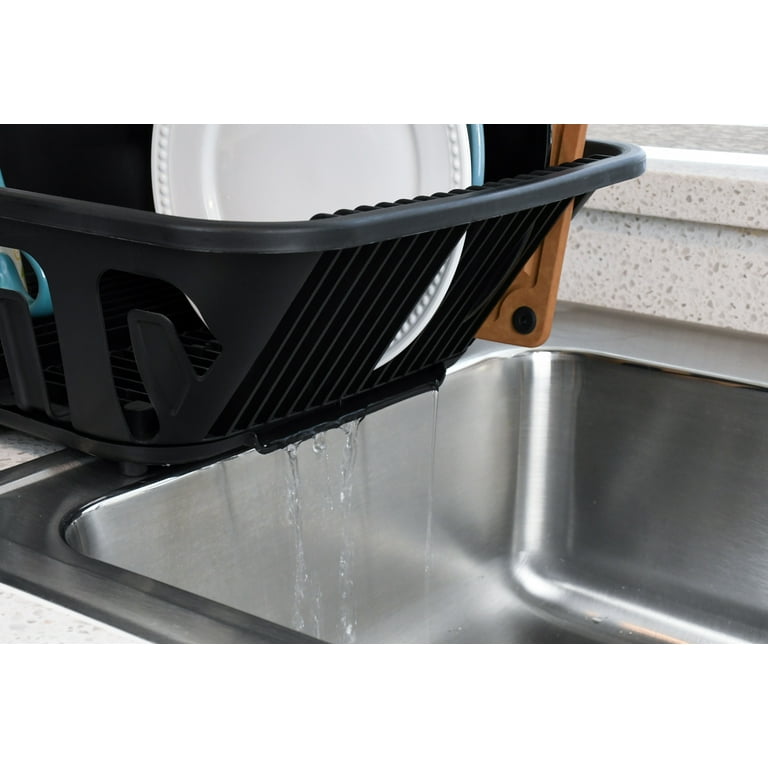This indoor photograph, set in a home’s kitchen, features a meticulous stainless steel kitchen sink with no visible signs of water or dirt. Positioned to the left of the sink is a black plastic dish rack, distinguished by its small feet that elevate it above the white counter speckled with gray and brown. The dish rack is thoughtfully angled to allow water to cascade off its right-hand side, dripping neatly into the sink. Within the dish rack, several dishes are visible: a large white dinner plate with a beveled edge, a blue dinner plate partially hidden behind the white one, and a black plate. A small rectangular wooden cutting board is also present, along with the handle of a mug slightly peeking out. The backsplash behind the sink appears to be a beige, spotted material, possibly tile or Formica, completing the clean and organized scene.